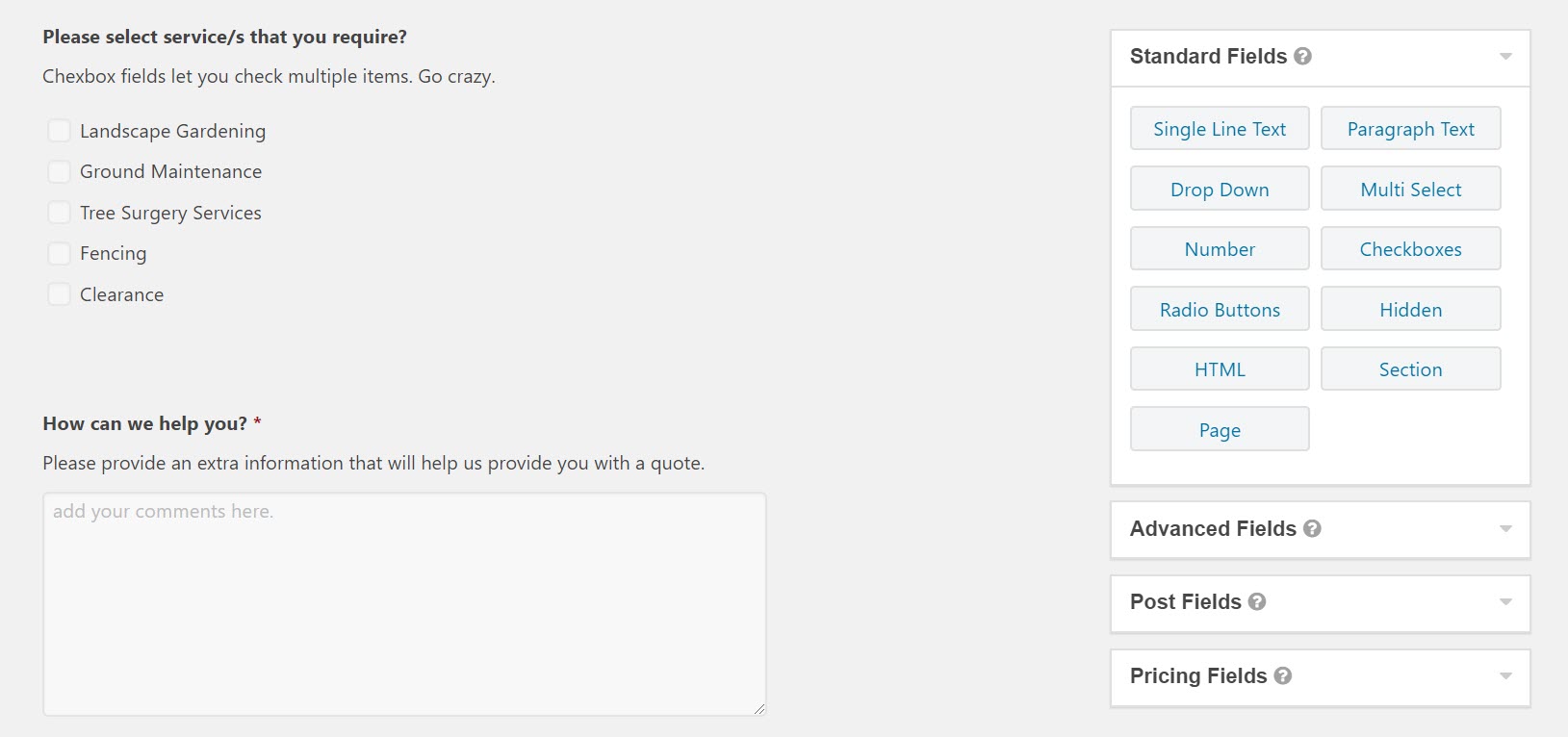This is a detailed screenshot of an administrative page for configuring a service request form. The central section prompts users with the header "Please select the service/services that you require," featuring checkbox fields that allow the selection of multiple service options. The five options listed are: Landscape Gardening, Ground Maintenance, Tree Surgery Services, Fencing, and Clearance. Below this section, a text prompts users with "How can we help you? Please provide any extra information that will help us provide you with a quote," followed by a large white input field labeled "Add your comments here."

To the right, there is a white panel with a green border titled "Standard Fields," containing a variety of buttons with blue text for adding form elements such as Single Line Text, Paragraph Text, Drop-down, Multi-select, Number, Checkboxes, Radio Buttons, Hidden HTML, Section, and Page. Below this, three additional options with drop-down menus are labeled "Advanced Fields," "Post Fields," and "Pricing Fields." Each of these sections is marked with a gray circle containing a white question mark, indicating help or additional information.

No options from the drop-down menus have been selected; only the standard fields at the top are active, as evidenced by the visible options in green and blue colors. The layout suggests that the elements on the left are what users will see on the public-facing site, while the right-hand elements are for customizing the visible options.